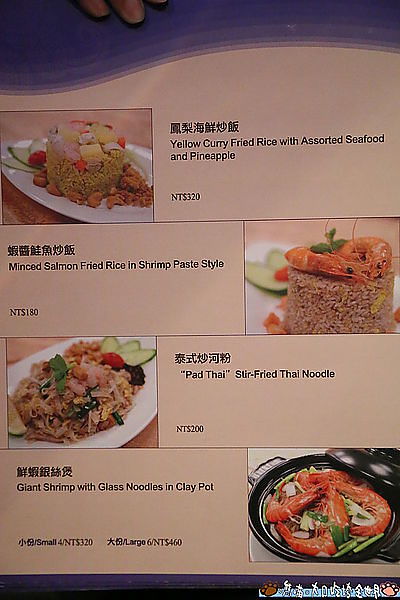The photograph is a page of a menu, predominantly white with a distinctive blue curved line at the top. It is divided into sections by black lines, each featuring tantalizing images and detailed descriptions of Asian cuisine. At the very top, partially visible fingers suggest the menu is laid flat on a table. 

The menu showcases four delectable dishes. The first, located in the top left, is a vibrant mound of rice adorned with assorted seafood and pineapple chunks, presented under the title "Yellow Curry Fried Rice with Assorted Seafood and Pineapple," priced at NT320. Adjacent to it, on the right, is an image of a rice dish garnished with two plump shrimp, labeled "Minced Salmon Fried Rice in Shrimp Paste Style," priced at NT180. 

Beneath these, on the left, lies a photograph of "Pad Thai Stir-Fried Thai Noodles," a plate brimming with noodles and a colorful assortment of vegetables and fruits, costing NT200. To its right, the final dish is "Giant Shrimp with Glass Noodles in a Clay Pot," featuring large shrimp atop a bed of glass noodles, priced at NT320. The captions indicate that the menu includes text in another language, likely Chinese, and a black stripe can be seen at the bottom of the menu.